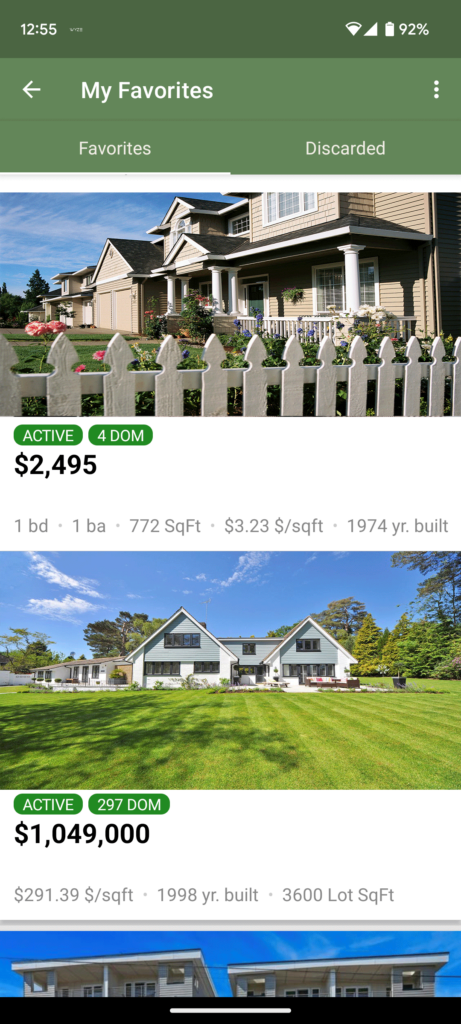This screenshot from a mobile phone displays a real estate listing with various interface elements and detailed property information. 

At the top, there's a leaf green status bar with white font: 

- The time is displayed in the upper left corner as "12:55".
- The upper right corner shows connectivity indicators: three out of four bars of Wi-Fi signal, full mobile signal strength, and a battery icon with "92%" next to it.

Below the status bar is a lighter green rectangle that reads "My Favorites" in white font, with a white, left-pointing arrow to the left of the text.

Further down, another green rectangle with white font displays "Favorites" and "Discarded." 

The main content features a picture of a two-story gray home with a built-on porch and a charming white picket fence in front of it.

Below the image, there are two small red ovals labeled "Active" and "For DOM," presumably indicating the listing's status.

The property listing details are provided beneath these indicators:

- The price is listed as "$2,495".
- In smaller gray font, the specifications mention the house has one bedroom, one bathroom, spans 772 square feet, and costs $3.23 per square foot.